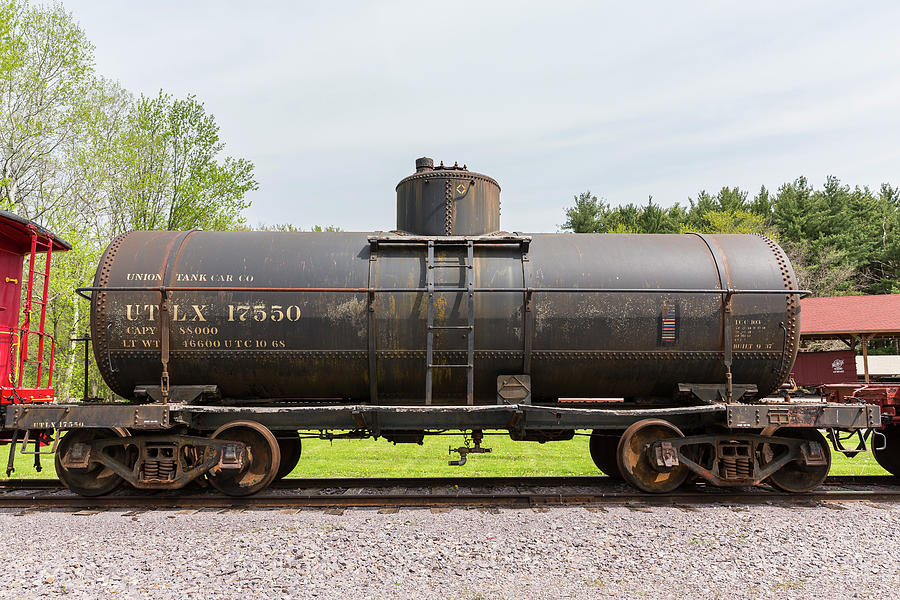This image captures an old, black cylindrical train tanker car, prominently marked with "Union Tank Car" and the code "UTLX17550" along its side. The tanker displays characteristic rust stains, particularly around its seams, and a central ladder with four rungs leading to a vent-like structure on top, indicative of its use for transporting liquid or gas. The train car rests on traditional, somewhat rusty wheels atop a track bed lined with gravel, interspersed with green grass on either side. It's a sunny day with a vivid blue sky dotted with wispy white clouds, and lush green trees form the backdrop, including birches to the left. In front of the tanker sits a red train car, though the details of the car behind it remain obscured.